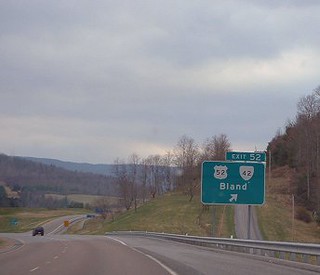A gray, overcast sky with heavy clouds looms over a multi-lane highway. The image prominently features a green exit sign edged in white, indicating Exit 52 for Bland with an arrow pointing to the right. The sign also lists Route 52 and Route 42 in white fonts against green medallions outlined in black. The highway surface is gray asphalt, marked with white lines, and fringed by a silver metal guardrail on the right. Several vehicles, including a black car, are spread across the highway. The right side of the image shows an additional smaller asphalt road with patches of green and brown grass and leafless trees, indicating the arrival of autumn. In the background, rolling hills blanketed with more naked trees add depth to the scene. Farther away, additional road signs in green and yellow are visible, complementing the expansive mountainous and wooded landscape.